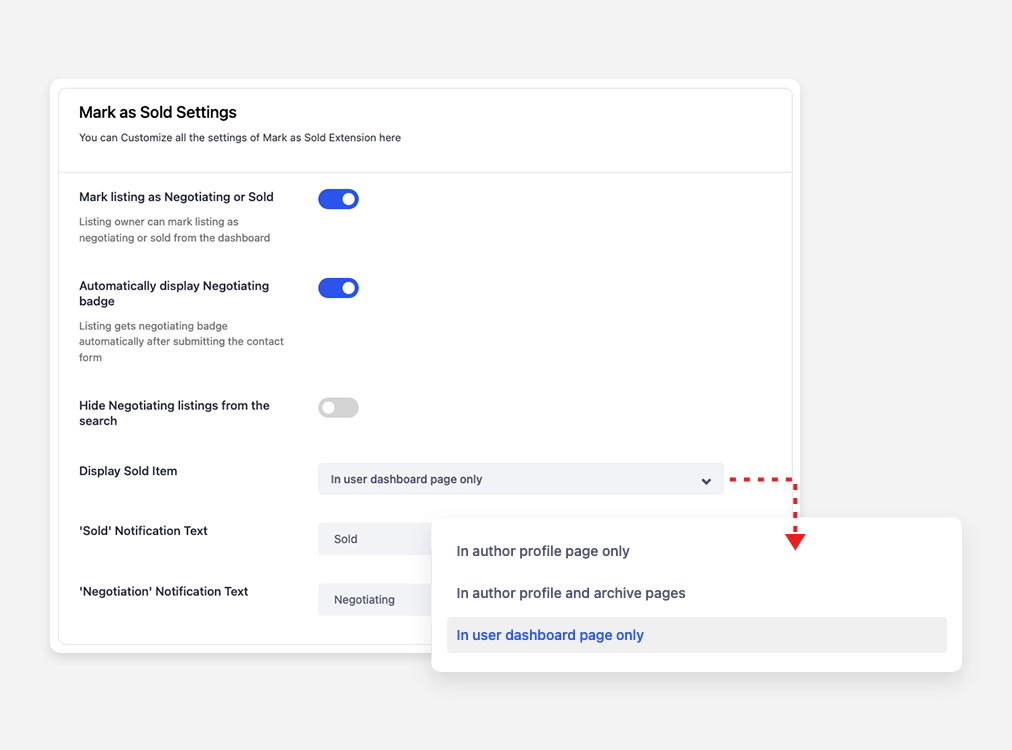Screenshot of a light gray interface featuring two pop-up white windows displaying settings. The first window, titled "Mark as Sold Settings," outlines various customization options for marking listings as sold or negotiating. The toggle button for "Mark listing as negotiating or sold" is enabled, allowing the listing owner to update statuses from the dashboard. Additionally, the "Automatically display negotiating badge" option is activated, resulting in listings automatically receiving a negotiating badge upon submission of the contact form. The "Hide negotiating listings from the search" option is disabled. Under "Display sold item in user dashboard page only," a drop-down menu is present, which is currently set to "In user dashboard page only."

A red dotted line with an arrow highlights the second pop-up window, which includes options such as "In author profile page only," "In author profile and archive pages," and "In user dashboard page only," with the latter being selected. On the left side of the interface, further settings detail notification texts associated with the sold and negotiating statuses.

The image is entirely textual, with no photographic elements, people, animals, or automobiles depicted.